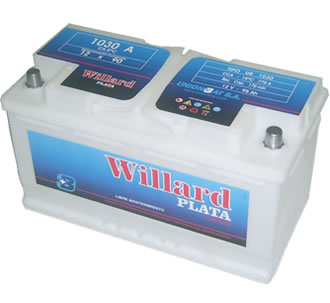The image depicts a white, plastic box-like device that strongly resembles a traditional sulfuric acid car battery. The box has two silver terminals, one on the left and one on the right. The brand name "Willard Plata" is prominently displayed on the front; "Willard" is written in red and "Plata" in white against an ocean-blue background. Above this, the text "1030A" is visible, likely indicating the model number. Additional small text, difficult to decipher, is also present on the device. A distinct letter "B" with a star is seen at the bottom of the front side. The entire background of the image is solid white, with no other objects or context visible. The device likely functions as a 12-volt battery, suggested by the markings and overall design.